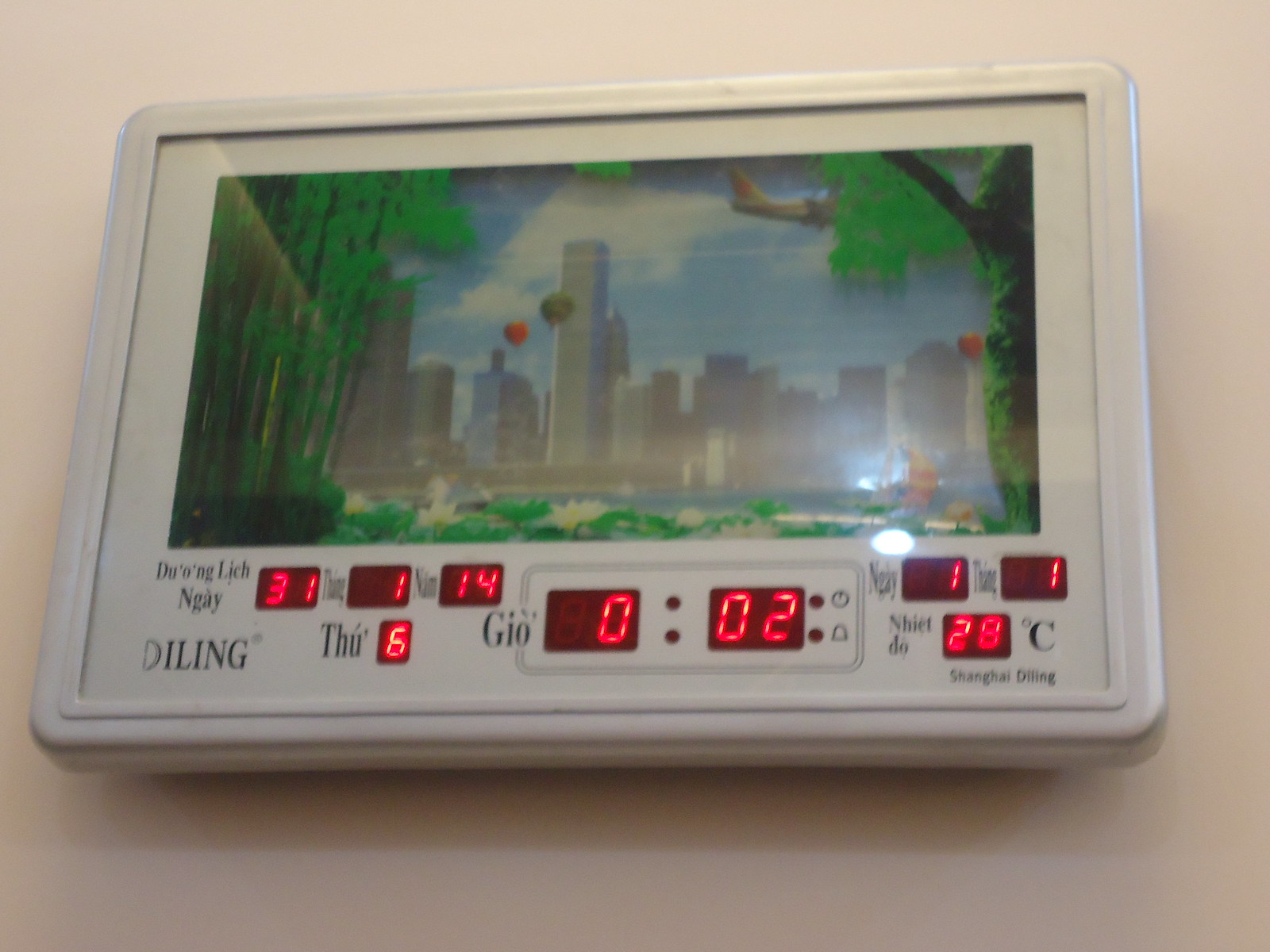A wall-mounted electronic device resembling either a thermostat or a timer is displayed. The unit, which is positioned against a cream-colored wall, is entirely labeled in Vietnamese. It features what appears to be a screen; however, it's unclear if this is a functioning digital display or a static image. The screen exhibits multiple functions, including a clock or alarm, a calendar set to January 31, 2014, and a thermostat, indicating the current temperature is 28 degrees Celsius. The specific functionalities beyond these are not discernible due to the language barrier.